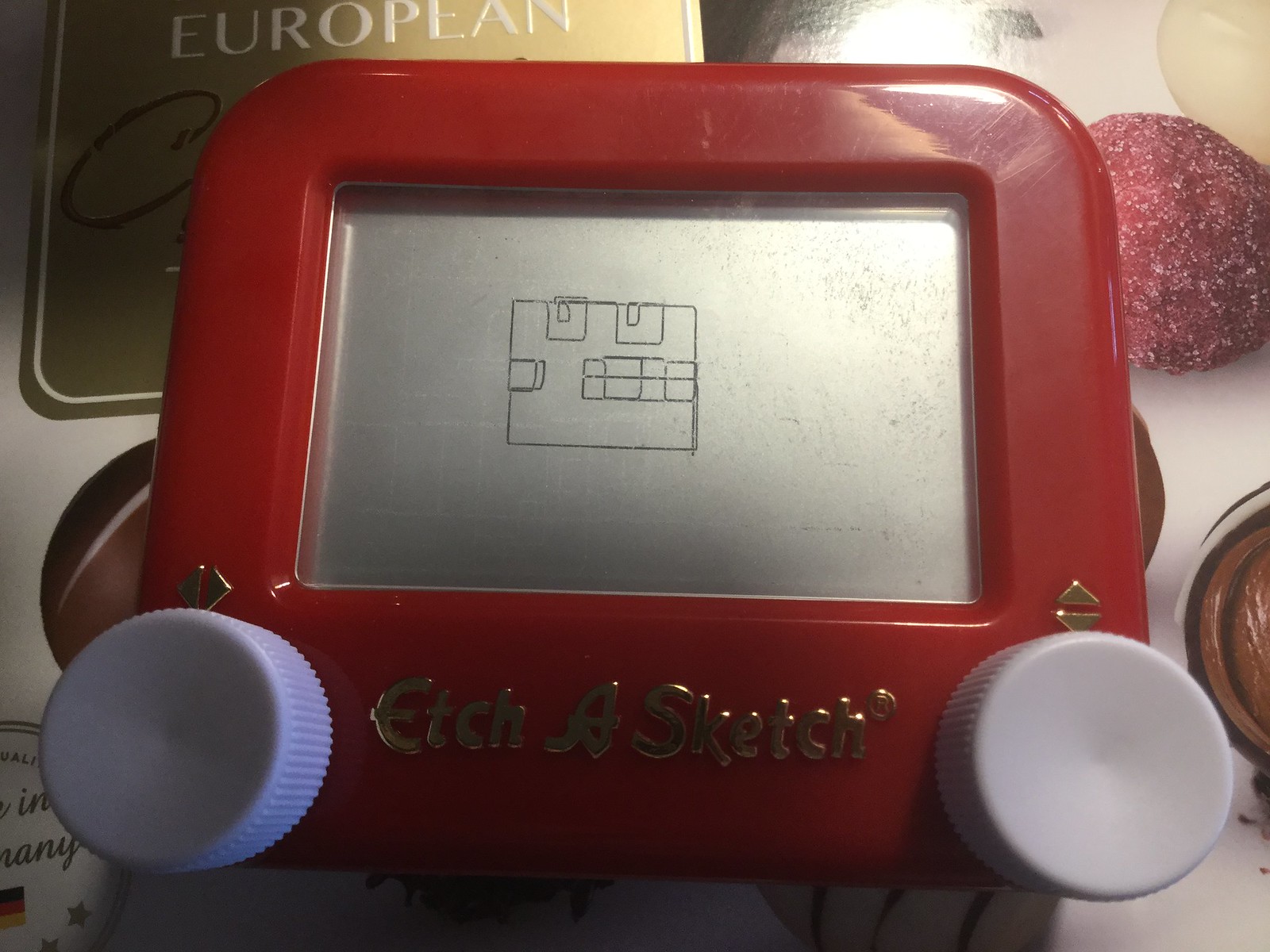This color photograph depicts a close-up view of a traditional Etch-a-Sketch, an iconic children's toy with a distinctive red plastic frame and two white circular knobs positioned at the bottom corners. Each knob is marked with arrows indicating the direction of drawing—left to right for the left knob and up and down for the right knob. The toy features a silver-gray screen where a drawing has been meticulously created. The primary image on the screen is a square-faced figure resembling a robot. The face includes square eyes, a mouth comprised of smaller squares and rectangles representing teeth, and additional squares to depict an ear on the left side. Below the screen, the name "Etch-a-Sketch" and its logo, including a registered trademark symbol, can be seen. The background provides a hint of the setting with several items visible: a gold advertisement with the word "European" prominently displayed, and various circular objects that are red, brown, and tan, likely representing sugary foods or decorations. The Etch-a-Sketch is set against an unclear surface, possibly a white table, adding to the nostalgic charm of the photograph.